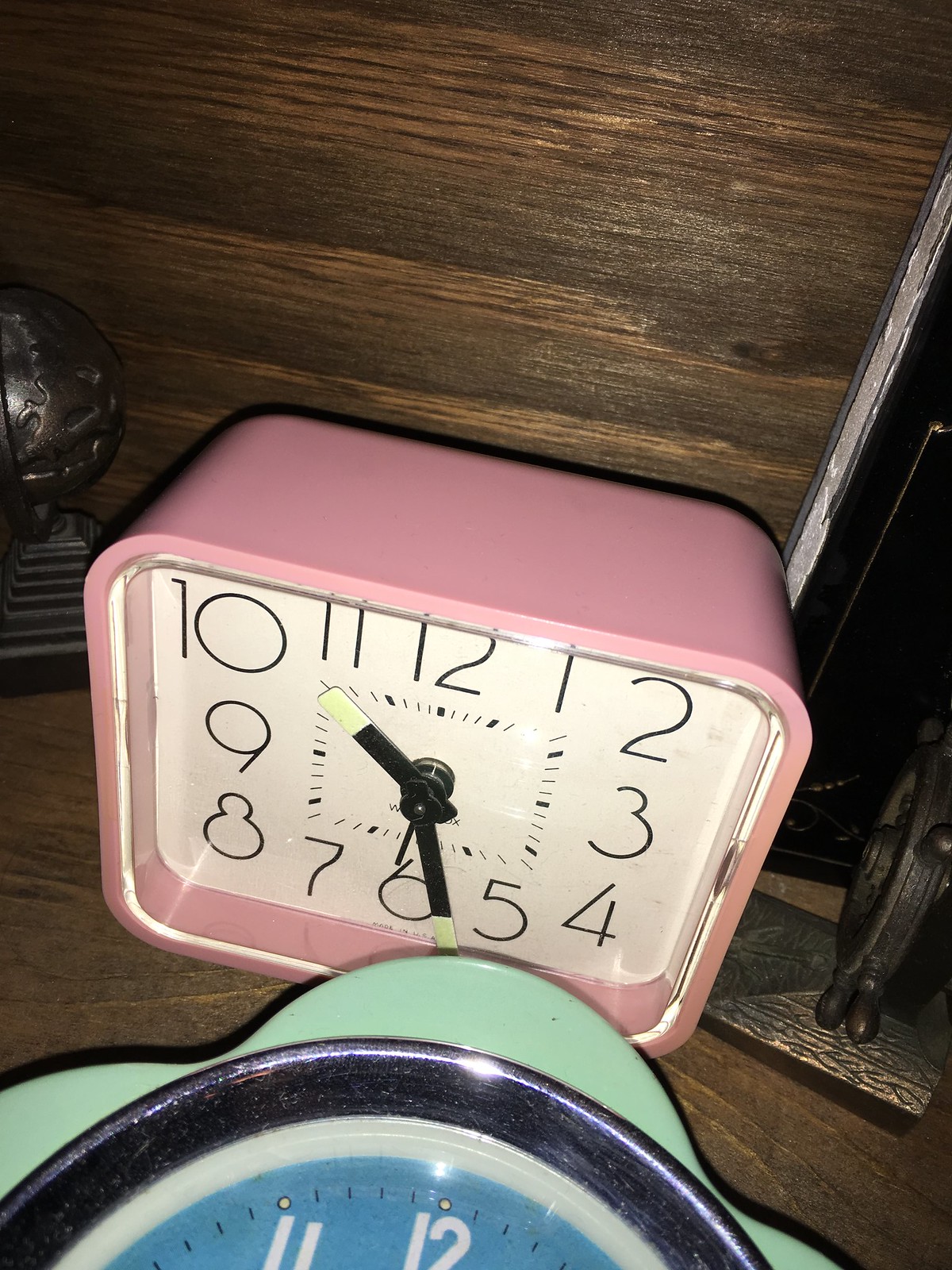In this detailed photograph, the main subject is a pink square alarm clock prominently positioned on a chocolate brown wooden table, which features a textured surface and matching wooden background. This pink clock is designed with a pink plastic case and a clear protective acrylic covering over the white clock face. The face displays large, rounded, modern black numbers from 1 to 12, surrounded by small black dashes indicating minutes, arranged in a square configuration inward from the numbers. The clock has an hour hand, a minute hand, and a slim second hand, all black with white tips that reflect green light at night. Set precisely at 6:15, this clock sits alongside two decorative bronze objects: a small globe on a step-pyramid base to the left, and a ship's steering wheel to the right. Both pieces are partially cut off by the edges of the frame but add a maritime theme to the scene. In front of the pink alarm clock, a smaller blue clock is partially visible. This secondary clock has a dark blue face with white numbers, an undulating light green edge, and a black and turquoise design framing its visible numbers, 11 and 12, which are mostly obscured by the pink clock. The overall image is a vertical rectangular shot, capturing the intricate details and positioning of these elements on the table.